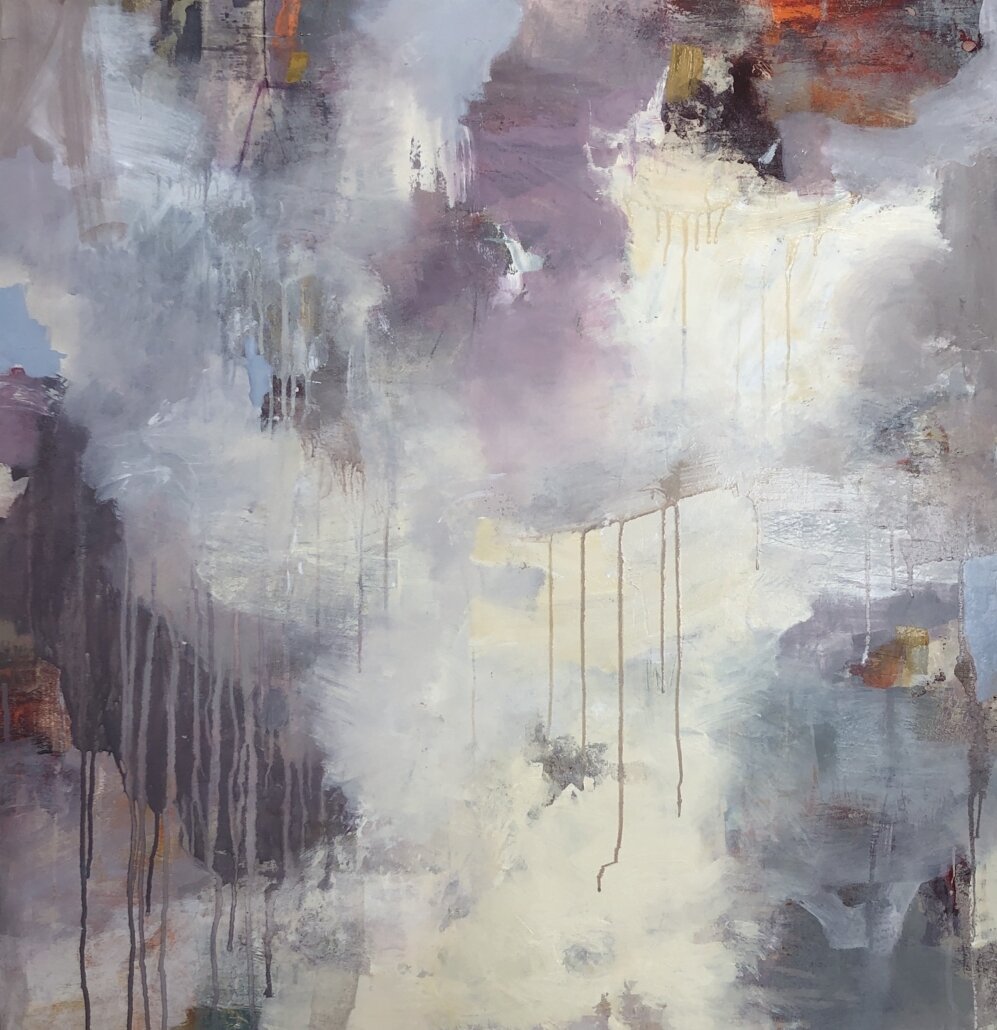The image is an abstract painting, perhaps created with a mix of watercolor and oil paints. The composition features various shades of gray, white, blue, purple, and occasional hints of red, yellow, and orange. The colors are distributed in cloudy splotches, patches, and dribbles, creating a somewhat chaotic and foreboding atmosphere. The splotches of color seem to simulate smoke or an explosion, with no discernible objects or text present. Vertical streaks of paint give the impression of drips, suggesting an organic and spontaneous creation process. The overall effect is blurry and obscure, with some areas showing through to a blue background. The painting contains a multitude of colors, including beige, black, deep purple, cream, and brown, layered on top of each other. The canvas seems to depict a scene of nebulous clouds or smoke, hinting at rain with drips and streaks symbolizing rainfall. It's a compelling piece that evokes a sense of abstract mystery and complexity.